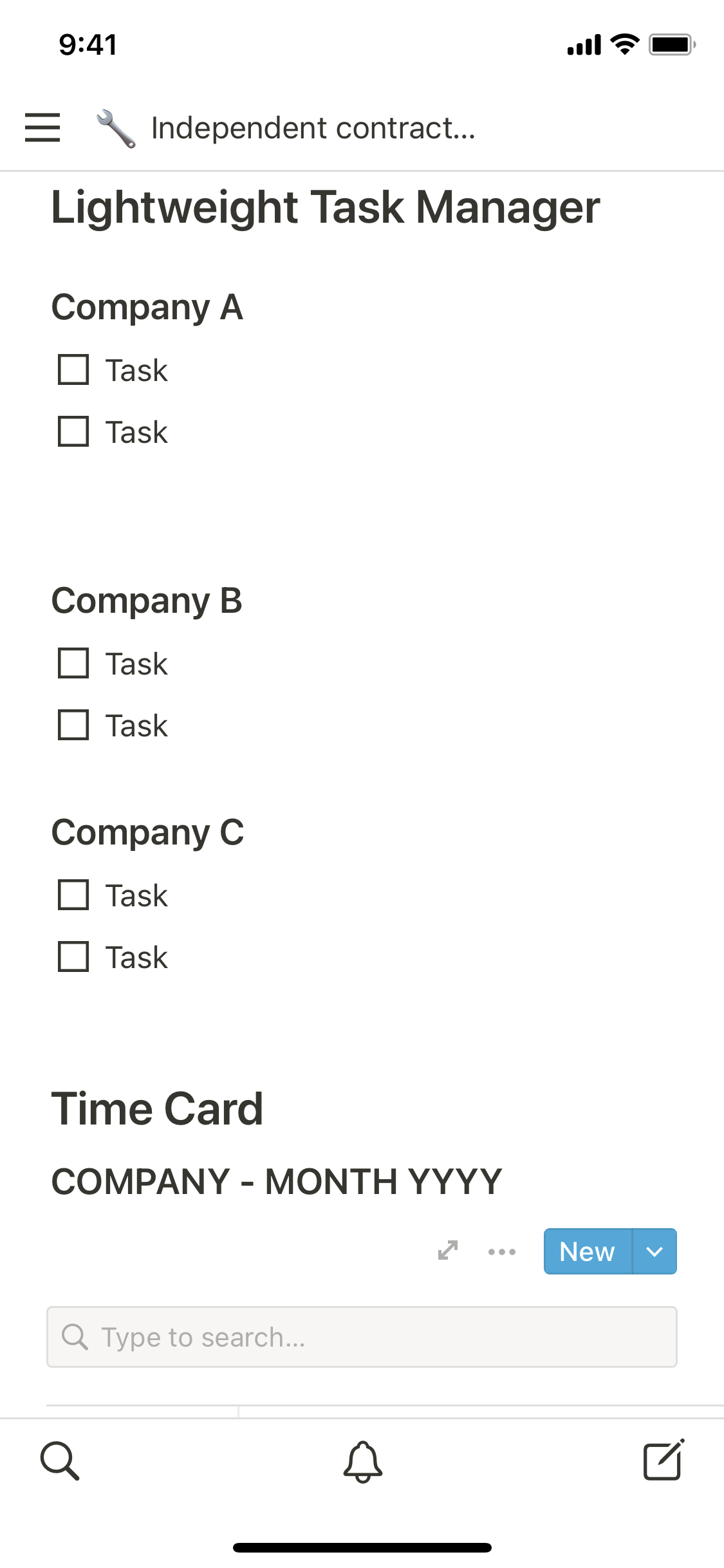This image is a detailed screenshot from a smartphone depicting a task management application designed for independent contractors. In the upper-left corner of the screen, the current time is displayed, flanked by the Wi-Fi signal indicator, battery life icon, and cellular service bars.

The background of the screen is white, providing a clean and minimalistic appearance. At the top of the application interface, there is a tool wrench icon followed by the text "Independent Contract" and "Lightweight Task Management" beneath it.

The application lists tasks associated with three companies: Company A, Company B, and Company C. Each company's section contains an assortment of tasks with checkboxes next to them. For Company A, there is one completed task marked by a checkmark in a box, and another task with an empty checkbox. Company B has two tasks, both with empty checkboxes. Similarly, Company C lists two tasks, each with an unchecked box.

Below the task sections, there is a "Timecard" page. Here, the display includes the word "Company" followed by a dash, and then a format placeholder for the date showing a month and "YYYY" for the year. Adjacent to this, there is a button labeled "New" for adding new entries. Directly beneath this button is a blank search box with the placeholder text "Type to Search" along with a magnifying glass icon, indicating the function to search tasks or entries.

At the bottom of the screen, three navigation buttons are visible. The first is a magnifying glass icon indicating a search function, the second is a bell icon representing notifications, and the third is a post-it note icon with a pencil, suggesting the option to create or edit notes or tasks.